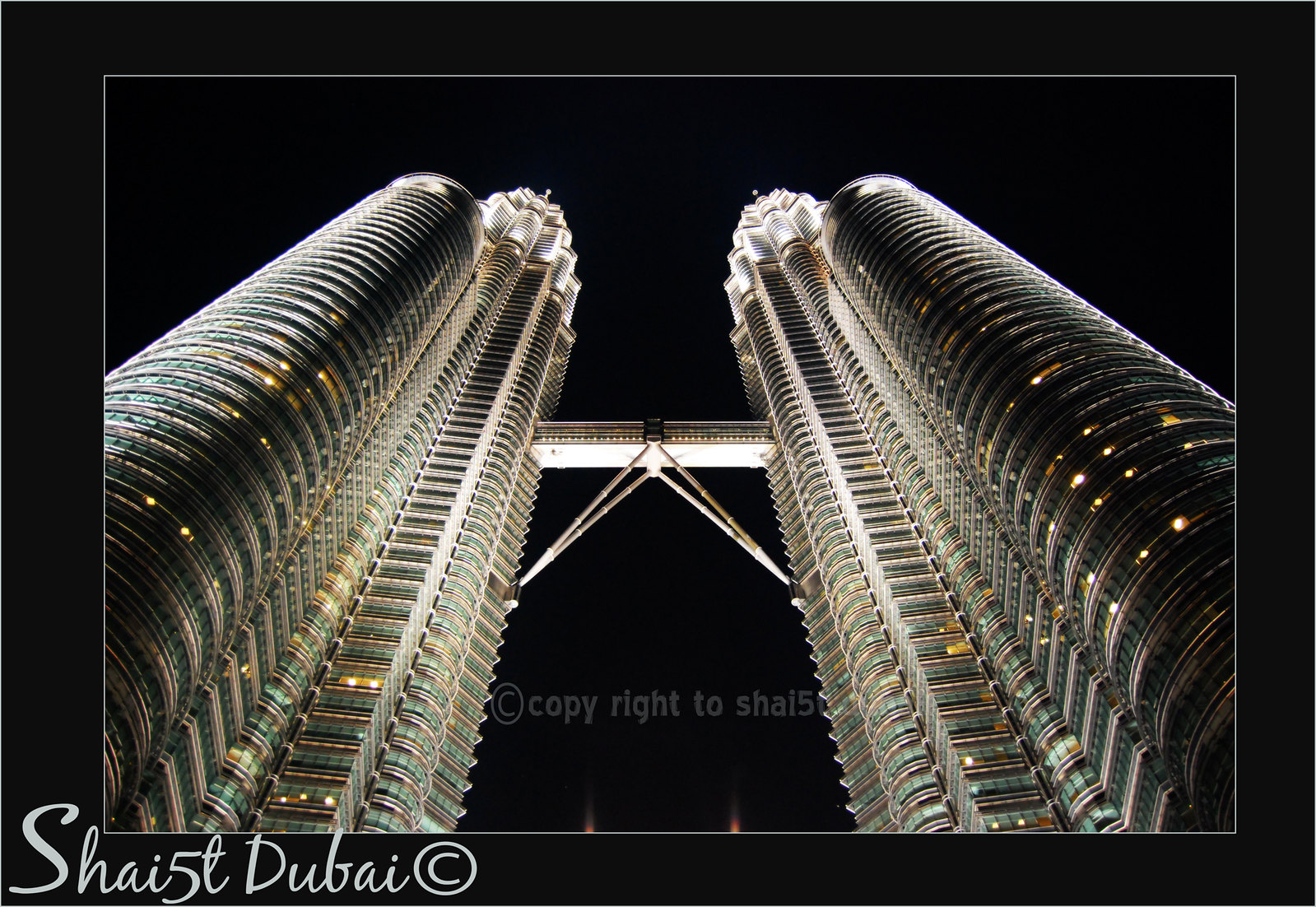The image depicts two towering skyscrapers, likely located in Dubai, framed within a dark black border with a thin white outline. A watermark in the form of a gray cursive script reading "Chi 5T Dubai" with a copyright symbol is placed on the bottom left and center bottom of the image. Both towers are identical, positioned on the left and right of the image, and are photographed from a low angle looking up into a dark night sky. The towers feature sparse lighting that intensifies towards their tops and are adorned with a mixture of greenish window reflections and metallic surfaces. A notable architectural feature of the buildings is a high-altitude aerial bridge connecting them, supported by two structural pillars extending from lower floors. This bridge appears to have windows along its span. The entire scene is visually punctuated by small lights at the base of the towers against the backdrop of the night.